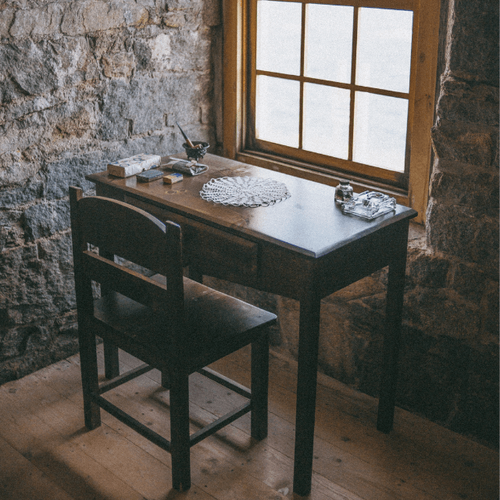This meticulously detailed color photograph, captured indoors during the daytime, offers a glimpse into a corner of a room. The image, square in shape and approximately four inches by four inches, showcases a scene rich in texture and contrast. The room features brown hardwood plank flooring that anchors the space with warmth. The walls are crafted from dark gray stone, visibly aged and characterized by lighter mortar and patches of orange discoloration due to wear.

In the upper right section of the photograph, a window punctuates the stone wall. This window, framed in brown wood casing, consists of six rectangular panes outlined by slender brown grid lines. Notably, the stone wall beneath the window shows increased signs of damage and erosion.

Central to the composition is a small wooden desk accompanied by a matching wooden chair, both angled slightly to give a three-dimensional impression. The desk, situated directly in front of the window, features a single drawer at its front. Atop the desk lies a circular white doily, an ink pot, and what appears to be an old pipe nestled inside a cup.

The style of the photograph leans toward representational realism, meticulously capturing the interplay of natural elements and man-made objects, offering a rich visual narrative that invites the viewer to ponder the history and utility of the depicted space.